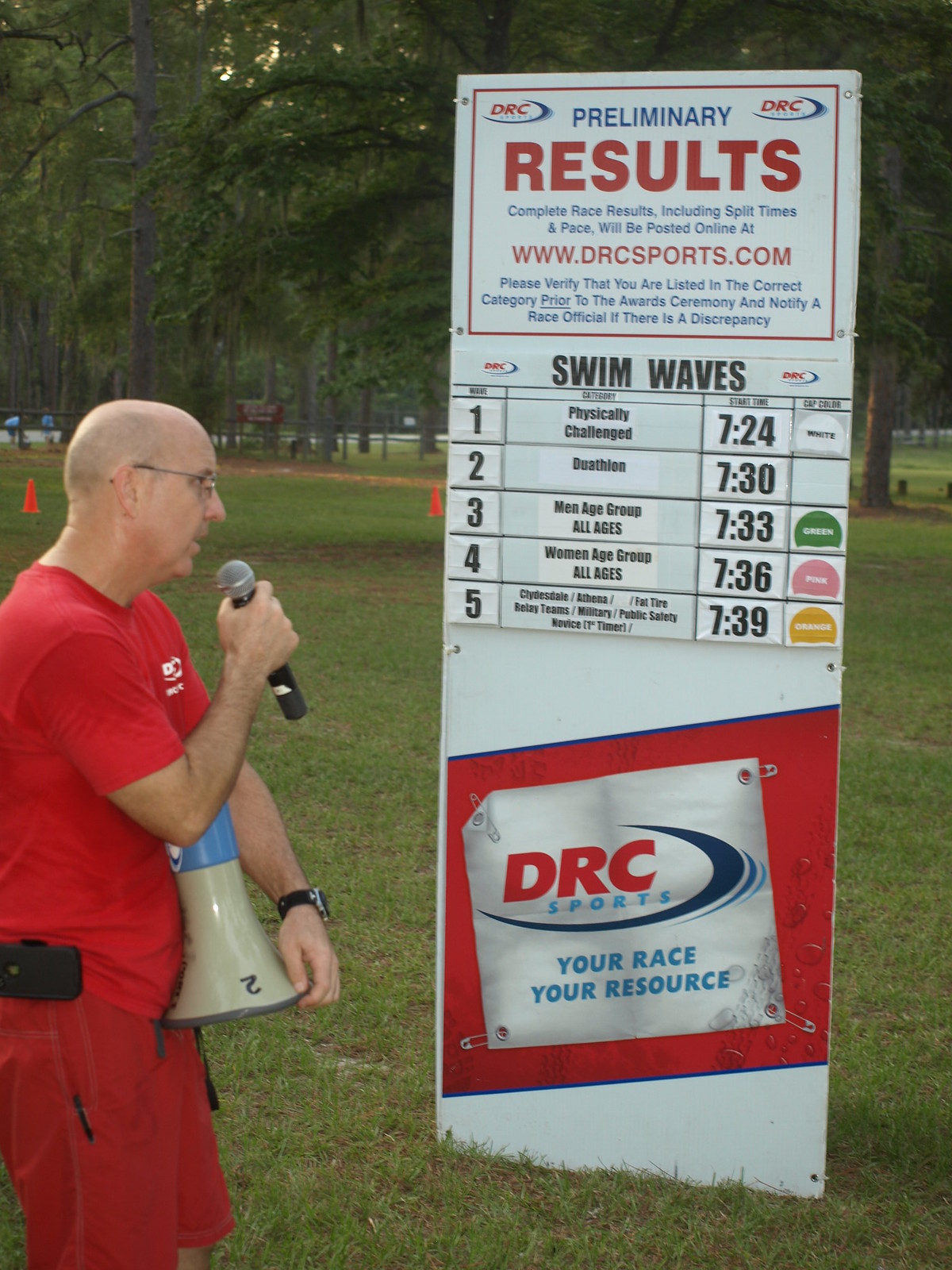The image is a vertically aligned rectangular photograph of a man standing outside in a green, grassy field with scattered tall trees in the background. The man, positioned on the left side of the picture, is bald on top and wears wire-rim glasses. Clad in a red t-shirt and red shorts, he has a black watch on his left arm and a cell phone holder clipped to his waist. The man's right arm cradles a light blue and tan bullhorn against his stomach while he speaks into a black microphone with a silver top held in his left hand. 

He is looking towards a large standing sign on his right, which features a white background framed by a red rectangular border. The sign prominently displays at the top "Preliminary Results", with "Preliminary" in blue letters and "Results" in large red, all-capital letters. Below this heading, it reads "Swim Waves" in bold black letters. The sign is organized into several columns: the first column numbered one through five, the second column listing categories with "Physically Challenged" and "Decathlon" among them, the third column indicating times such as "724", and the fourth column displaying color-coded text like "white", "green", "pink", and "orange". At the bottom, the sign contains an area displaying "DRC sports, your race, your resource" alongside instructions to verify category listings and ensure accuracy. Safety cones can also be seen dispersed in the background, indicating an organized event space.